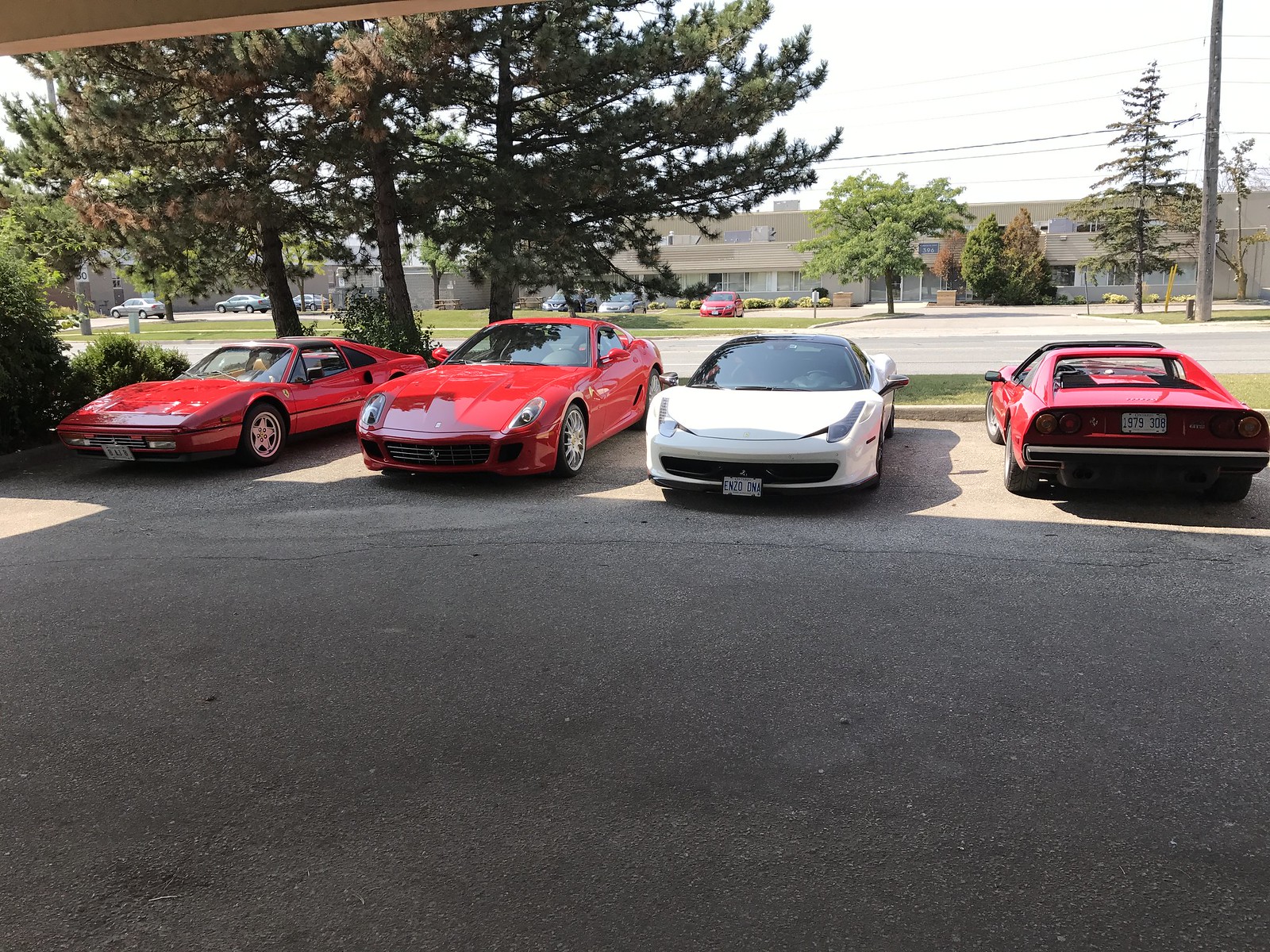This photograph, taken outside, captures a line of four classic exotic sports cars from the 1980s and 1990s parked in a parking lot. Three of these cars are bright red, and one is white. Starting from the left, the first car is a red sports car, possibly a Corvette. Next to it is another red sports car, perhaps a Porsche. The third car is a white sports car, while the fourth on the far right is another red sports car, which is the only one facing away from the camera, showing its back. 

All these cars appear to be Ferraris in varied models, with the older versions placed at the extreme ends and the comparatively newer versions in the middle. The lot is partially shaded by nearby trees. Beyond the small strip of grass and trees that line the lot, there is a road. On the opposite side of this road stands a two-story office or school building with brown walls and rectangular windows. The building's parking area also contains several parked cars that do not seem to be sports cars.

The background scenery includes several trees, including some pines, and a telephone pole to the right side of the image. Overall, the setting gives the impression of a car meetup or a casual display of these vintage exotic vehicles in an open, spacious parking lot that extends over an asphalt ground.